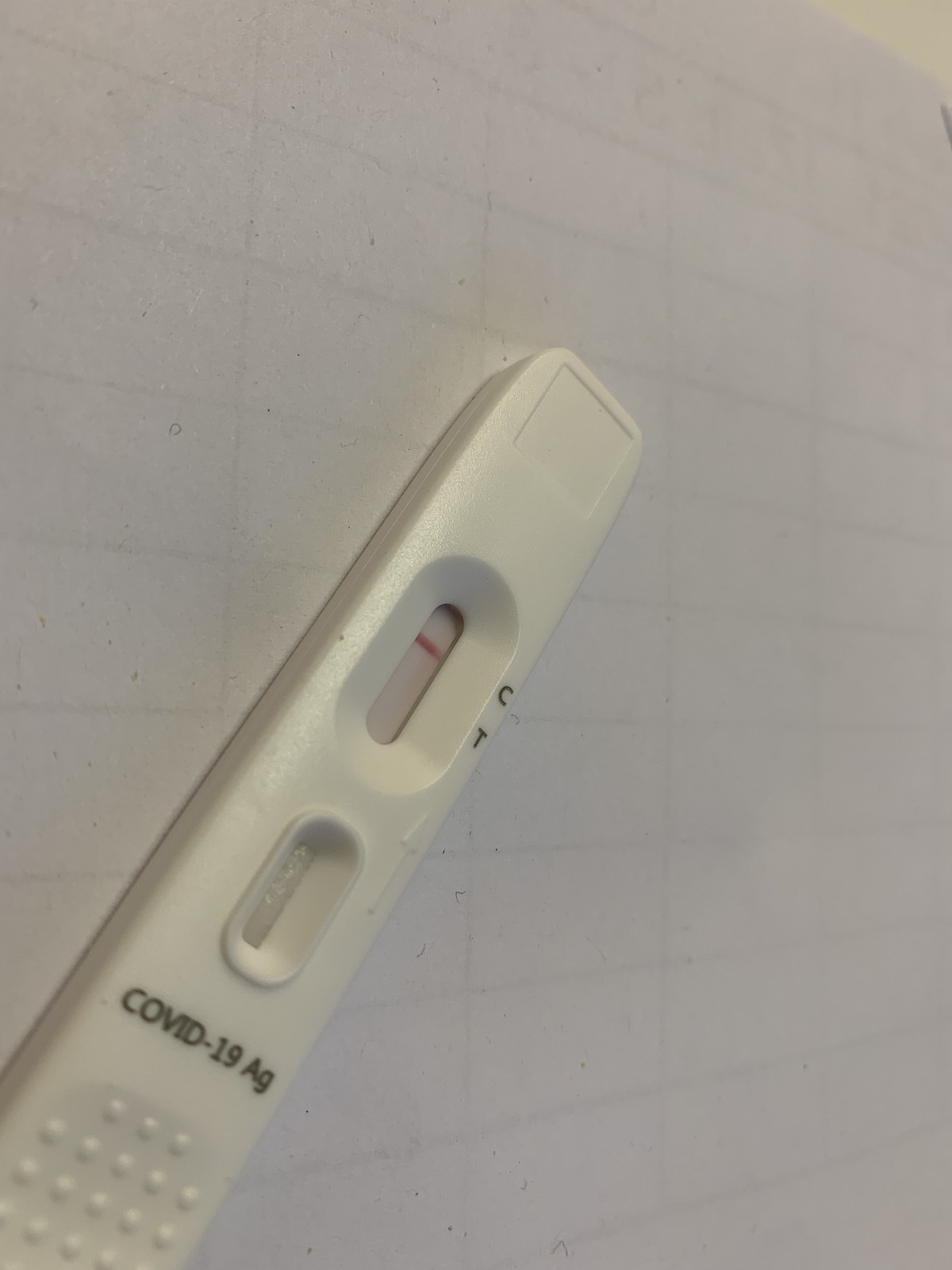The photograph captures a COVID-19 at-home testing kit placed in an indoor setting. The test device, predominantly white in color, prominently features distinct labels on the side marked as 'C' and 'T'. Positioned at the bottom of the test, bold black letters spell out 'COVID-19 AG'. A noticeable white line is visible next to the letter 'C', indicating the test's status. The background features a collection of neatly stacked rectangular objects, all uniformly white, creating a clean and organized appearance. The entire image is framed within a rectangular shape, emphasizing simplicity and clarity.